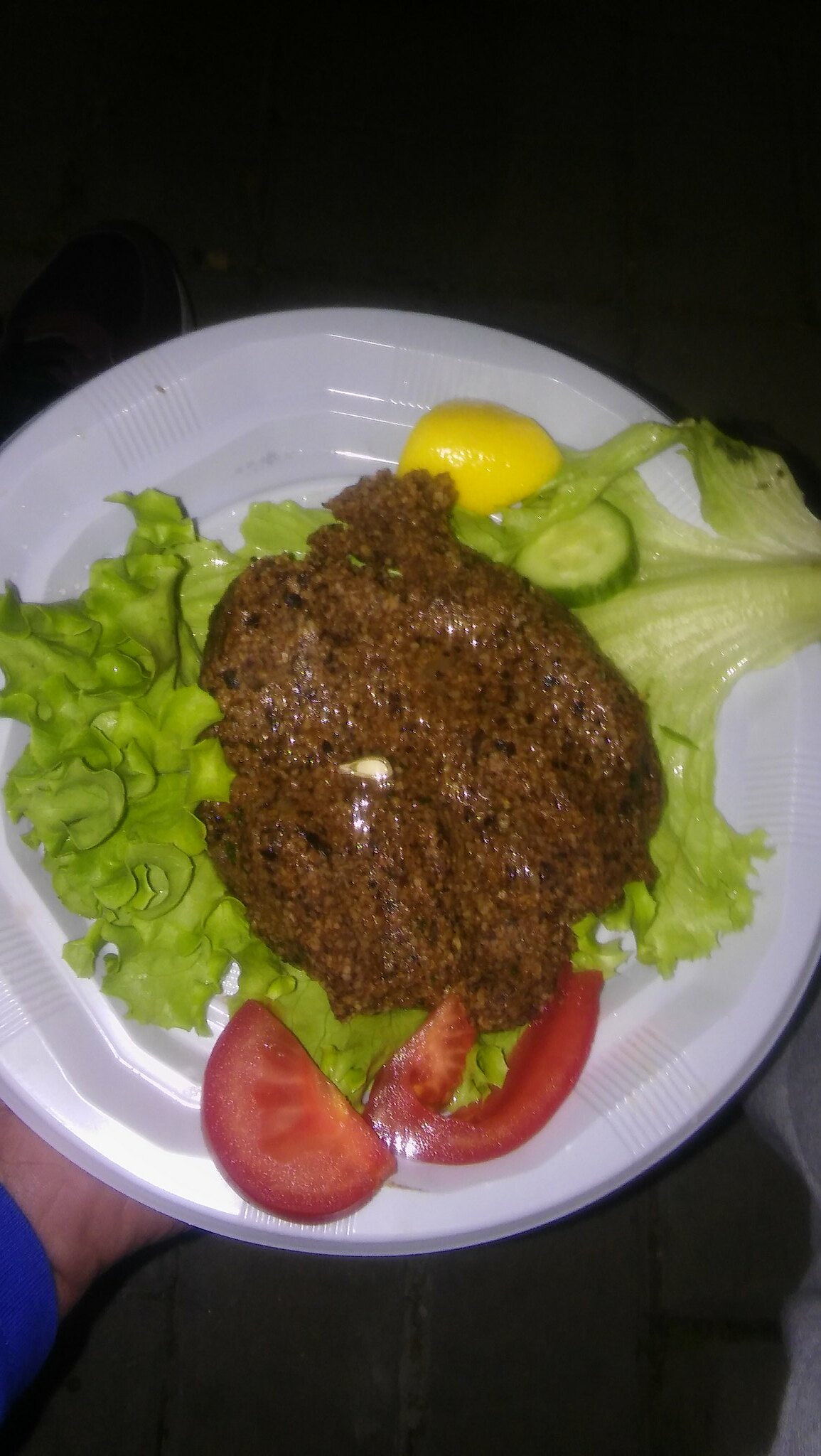The photograph is a rectangular image set against a completely black background, taken in low lighting which gives the scene a dark and intimate feel. It captures a person's left arm extending slightly to display a sturdy white styrofoam plate. The plate is adorned with a carefully prepared dish that seems to be a bunless burger. A large, crisp green leaf of lettuce serves as the bed upon which sits a hand-formed, irregularly shaped brown patty, adorned with small black speckles and possibly a seed. Surrounding this central meat piece are fresh, vibrant vegetable garnishes: a wedge of bright yellow lemon, a couple of thin cucumber slices, and two rich red tomato slices tucked beneath the patty. Only a glimpse of the person's wrist is visible, clothed in the royal blue cuff of their shirt, adding a pop of color to the otherwise dark scene. The positioning suggests the photo might have been taken with the plate resting on the person’s lap, adding an informal, candid touch to the setting.